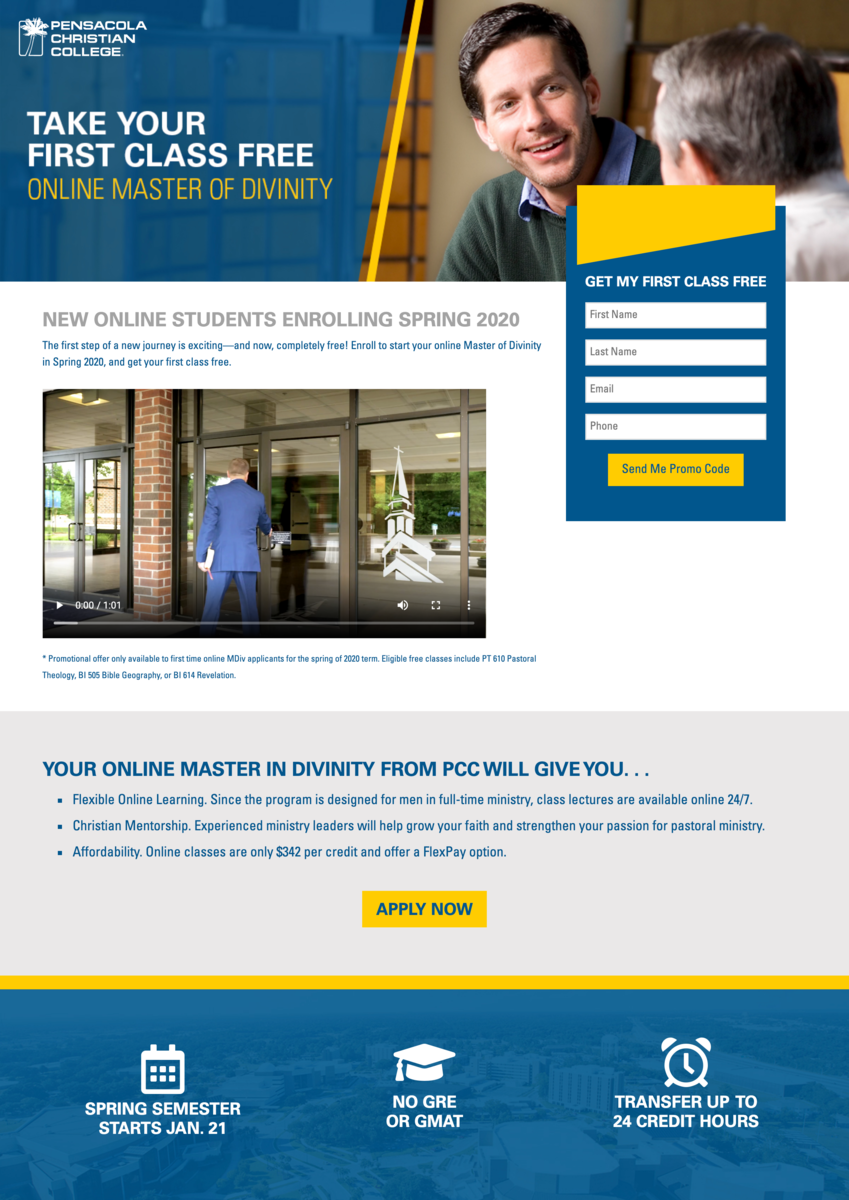The image is an advertisement for Pensacola Christian College, prominently featuring their logo and branding in the top left corner in white. Bold white text beneath the logo announces, "Take your first class free," promoting their Online Master of Divinity program. 

To the right, an indoor photograph captures a moment between a younger man, who is smiling and engaged in conversation, and an older man, whose back and side profile are visible. 

Below this image, text indicates, "New online students enrolling Spring 2020." Adjacent to this, there’s a photograph of the exterior of a brick building with numerous windows. A person is shown opening the door, seemingly about to enter.

Further to the right, there is a sign-up box inviting prospective students with the heading, "Get my first class free." The box contains four fields for first name, last name, email, and phone, followed by a button labeled, "Send me promo code."

Further down, a blue text box outlines the benefits of earning an online Master of Divinity from PCC, listed with three bullet points: 
1. **Flexible online learning:** The program is designed for men in full-time ministry, with class lectures available online 24/7.
2. **Christian mentorship:** Experienced ministry leaders will help grow your faith and enhance your pastoral ministry skills.
3. **Affordability:** Online classes are offered at $342 per credit with a flexible payment option.

At the bottom, an orange button encourages immediate action with the prompt, "Apply now."